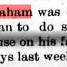This image is incredibly small, about half an inch on each side, making the text difficult to decipher. It features a partial display of text spread over four lines. In the upper left corner, the text "A-H-A-M" is highlighted in red, followed by the word "WAS." Adjacent to this is a sequence that reads "A-N-2-D-U-S." Below, there appears to be an incomplete phrase "S-E ON HIS F," with a black or dark highlight. The final line at the bottom has partial words "Y-S," "LAST," and "W-E-E," likely meant to form "WEAK." The text is displayed against a white background, further complicating the identification of the complete content. The image seems to capture only fragments of a larger text, leaving its full context unclear.